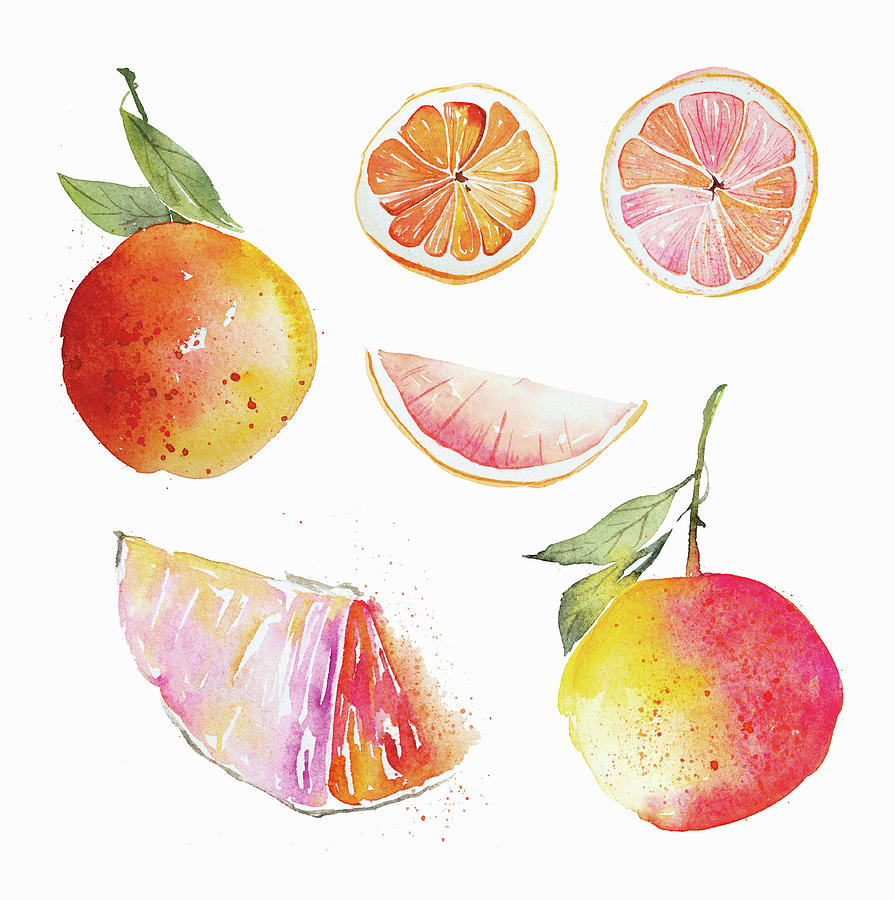This image is a detailed watercolor illustration of various forms of what appears to be oranges with a white background. The composition includes six distinct pieces of fruit. At the top, there are two cross-sections of oranges, displaying their juicy, segmented interiors. To the left, there is a whole fruit that closely resembles a peach, featuring a peach-colored skin with red speckles and two green leaves. In the middle, a vibrant pink slice likely represents a grapefruit. The bottom left showcases a peeled grapefruit slice, bitten in half, with a reddish interior and a purple-yellow exterior tint. Lastly, in the lower right corner, there is another whole fruit with yellow and slightly pinkish hues, accompanied by two leaves, possibly indicating it's another variation of an orange or peach. The illustration uses abstract and vibrant colors, making the identification of each fruit uniquely expressive yet somewhat ambiguous.